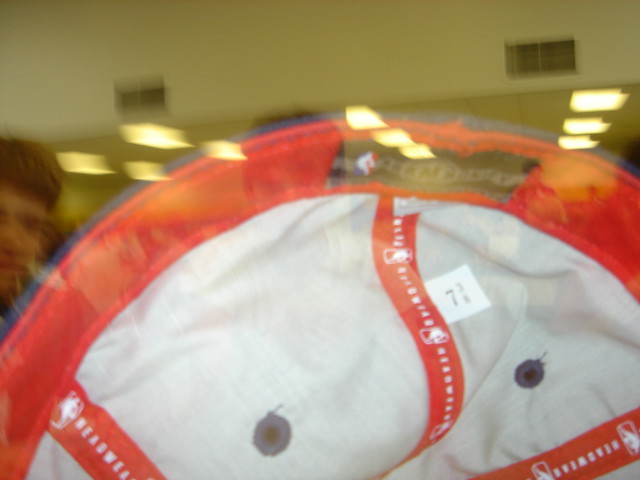In the image, a blurred man with brown hair is positioned on the left side, facing the camera. He appears to be holding a red and white object that looks deflated and difficult to identify; it may have some connection to the NBA based on visible licensing symbols. The object could initially be mistaken for a tent due to its striped pattern, but the NBA symbol suggests it is more likely sports-related. The background features a yellow ceiling adorned with numerous lights and scattered air vents, adding to the indoor ambiance of the scene.